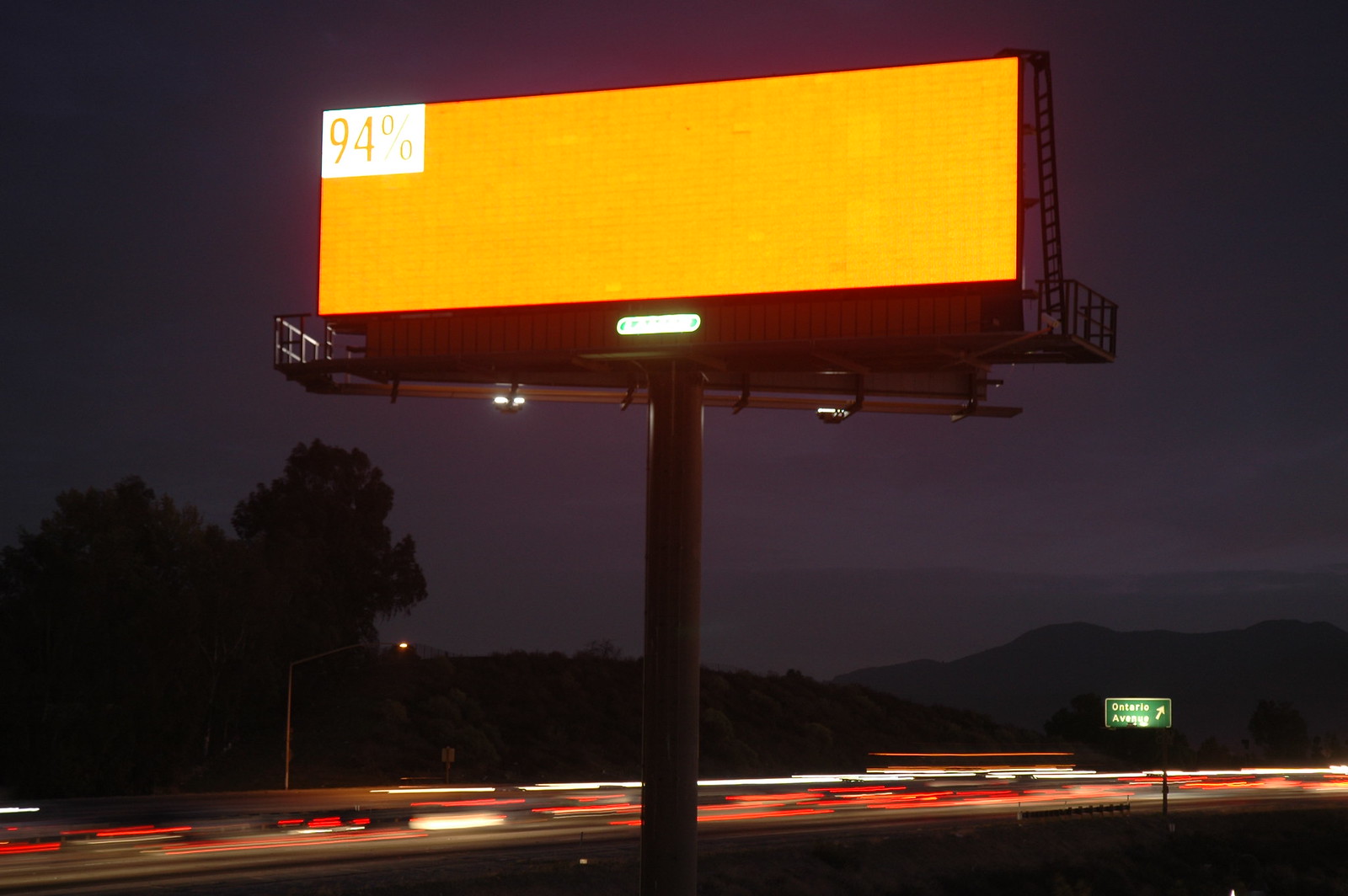This nighttime photograph captures an expansive landscape dominated by a large, brightly-lit, orange billboard mounted on a black metal pole. The billboard's orange display is three times wider than it is tall and features the text "94%" in the upper left corner, set against a white background. A grayish sky, tinged with deep purple hues, hints at a time just after sunset. The horizon, marked by the silhouettes of a tree line and a mountain range, frames the scene. Below the billboard, a highway is visible, with streams of red and white light indicating long-exposure captures of taillights and headlights. The left side of the image shows the traffic more clearly, while a green highway exit sign, potentially for Ontario Avenue, is seen towards the bottom right. The billboard also features a metal walkway and stairs leading up to the top, and a dark letterbox at the bottom with an indistinct green logo at the center.